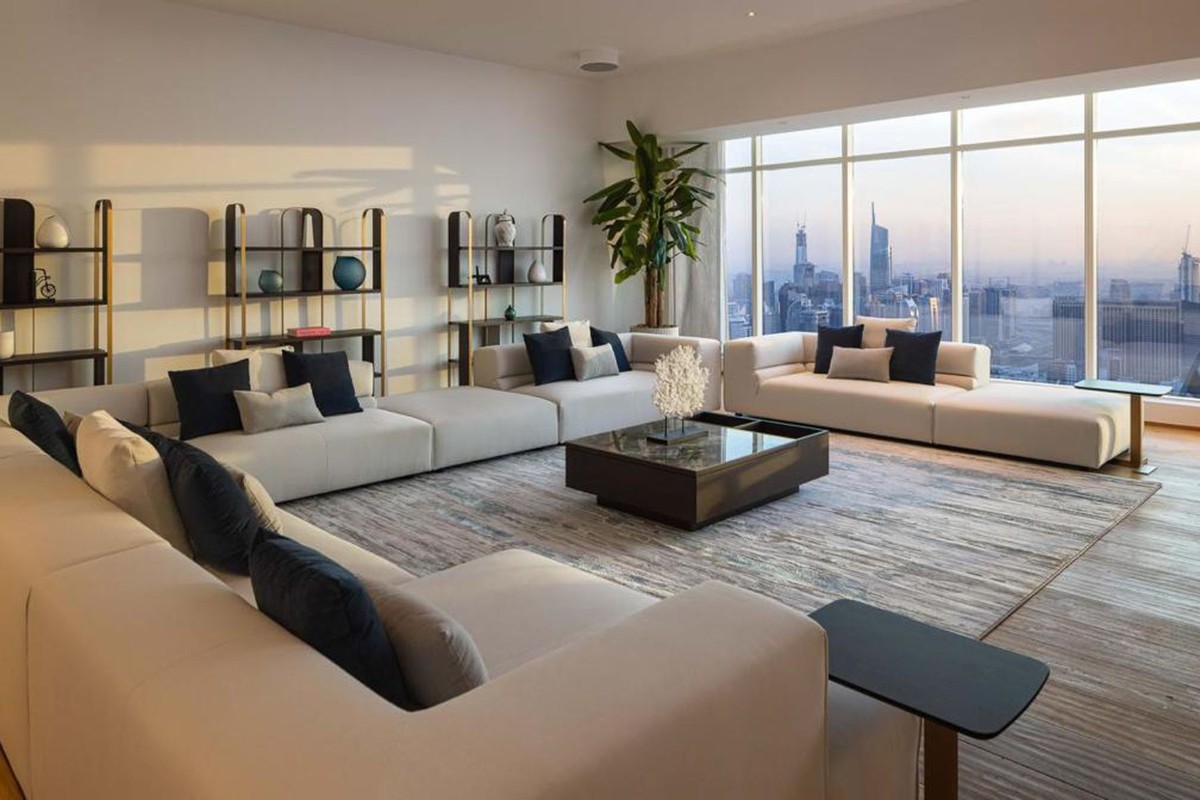This indoor photograph, likely taken in an apartment building in a bustling city such as New York or Chicago, showcases a spacious, well-furnished living area. Central to the room is a black coffee table with a glass top, which features a decorative miniature tree. The table’s drawer is open and faces away from us. Arranged in a C-shape along the room’s perimeter is a series of cream or beige sectional sofas adorned with cushions in black, beige, dark blue, and gray hues. 

A floor-to-ceiling window on the right side of the photo provides a stunning backdrop of various skyscrapers, suggesting a high-rise urban setting. The sky visible through the window appears yellowish near the horizon and lighter above, indicating the photo was likely taken at sunrise. Next to the window, a white potted plant with thick green leaves adds a touch of nature to the scene. Against the left wall, a set of three shelves are filled with knickknacks, providing additional character to the room. Overall, the space combines modern decor with a cozy, lived-in feel.